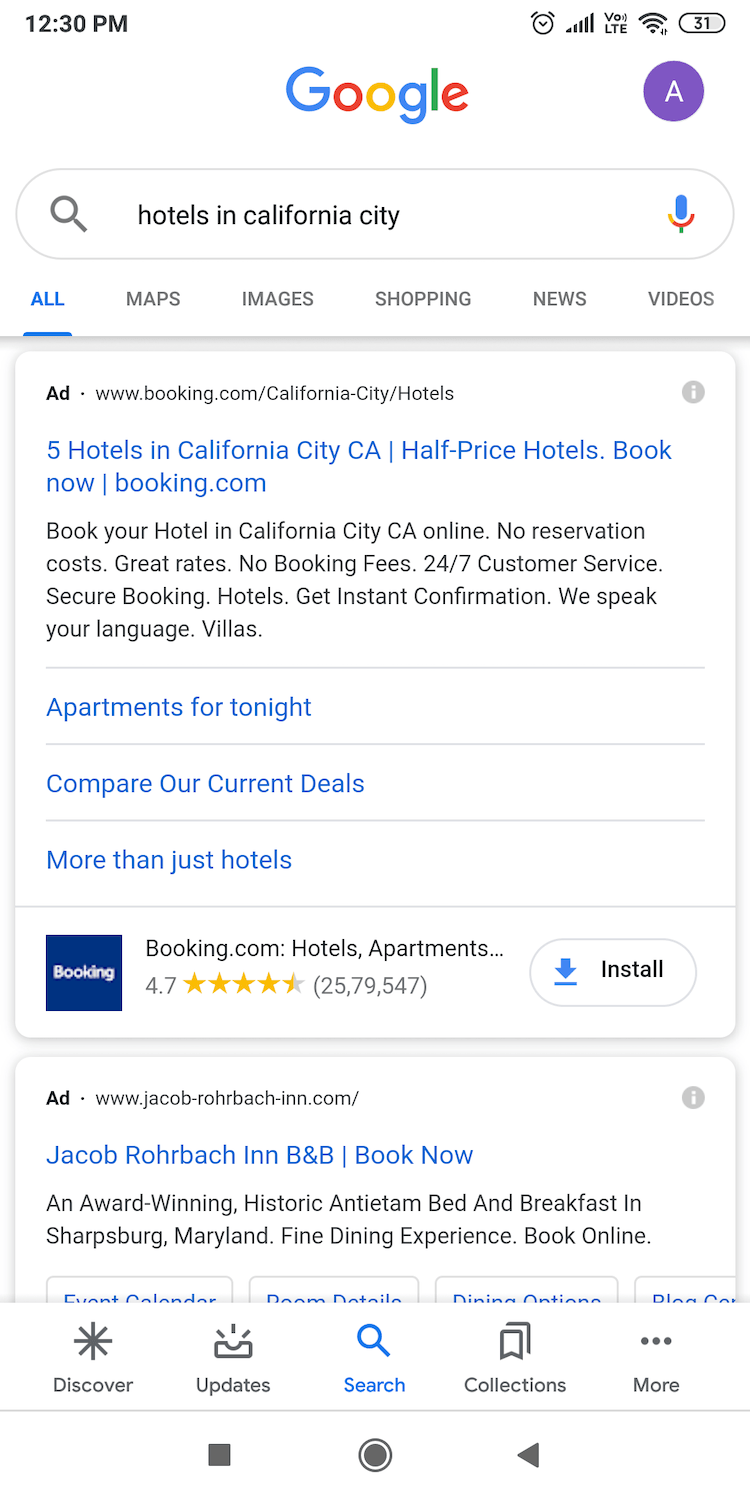The image depicts a Google search webpage displayed on a smartphone screen. The phone's battery is at 31%, and the device indicates a strong 4G LTE connection at 12:30 p.m. The Google logo, featuring its signature blue, red, yellow, and green colors, is prominently visible at the top. To the upper right corner, there is a purple square icon with a white 'A' inside.

Under the Google search bar, which includes a microphone icon, the user has typed "hotels in California City," highlighted in blue. Below this search query, the search results show: "5 hotels in California City, California," along with promotional information from booking.com in blue text, urging visitors to "book now" for half-price hotels.

The results also state in black text that users can "book your hotel in California City, California online" with no reservation costs, great rates, and no booking fees. Another highlighted segment in blue reads: "apartments for tonight," encouraging visitors to compare current deals for "more than just hotels."

Further down, a blue booking icon with white lettering for "booking.com" appears, suggesting visitors can install the app, which boasts a rating of 4.7 stars. Mentioned is the "Jacob Robach Inn" bed and breakfast, which prompts the user to book now. The search results are truncated at this point, and the phone’s bottom icons are partially visible.